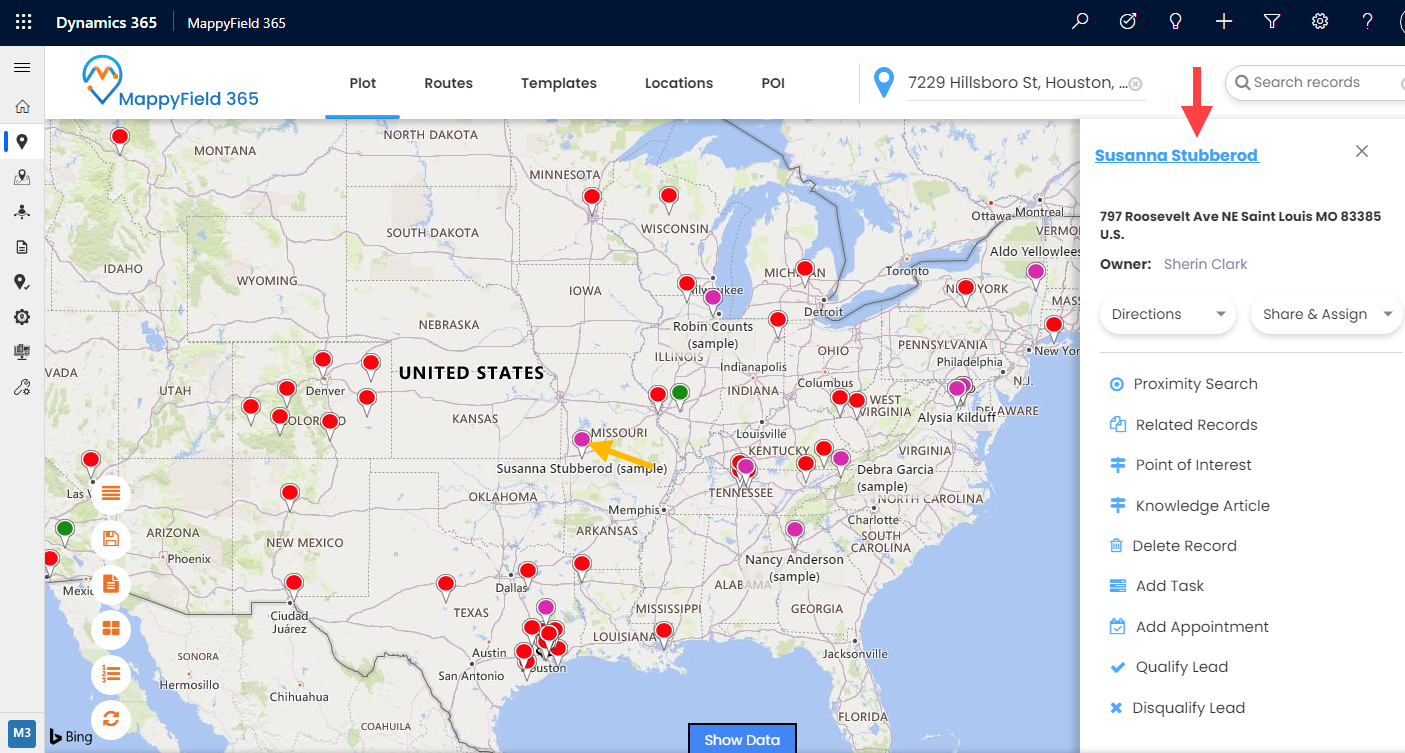This is a detailed image of a map from the MappyField365 website, prominently displayed with its logo and a menu bar at the top left corner. The menu includes options such as "Plot," "Routes," "Template Locations," along with an address bar and a "Search Records" bar. The focal point of the image is a map of the United States, featuring red and purple dots to indicate various locations. 

The red dots predominantly concentrate around Houston, Texas, and areas in Colorado, while the purple dots are clustered primarily around the Southeast and Mid-Atlantic regions. A legend is provided for reference, and a "Show Data" tab is located at the bottom. The map is sourced from Bing, with a Bing copyright notice at the bottom left side. 

Additionally, the map features a left sidebar populated with various icons and a right sidebar titled "Susanna Stubbard," detailing an address at 797 Roosevelt Avenue, Northeast St. Louis, Missouri. The section lists the owner as Sharon Clark and offers two interactive buttons: "Directions" and "Share and Assign." At the top of this sidebar, a red arrow points to the name Susanna Stubbard, which is formatted in blue and underlined. 

Below these buttons, there's a comprehensive list related to the map that includes functions like Proximity Search, Point of Interest, Delete Record, Add Task, and Disqualify Lead.